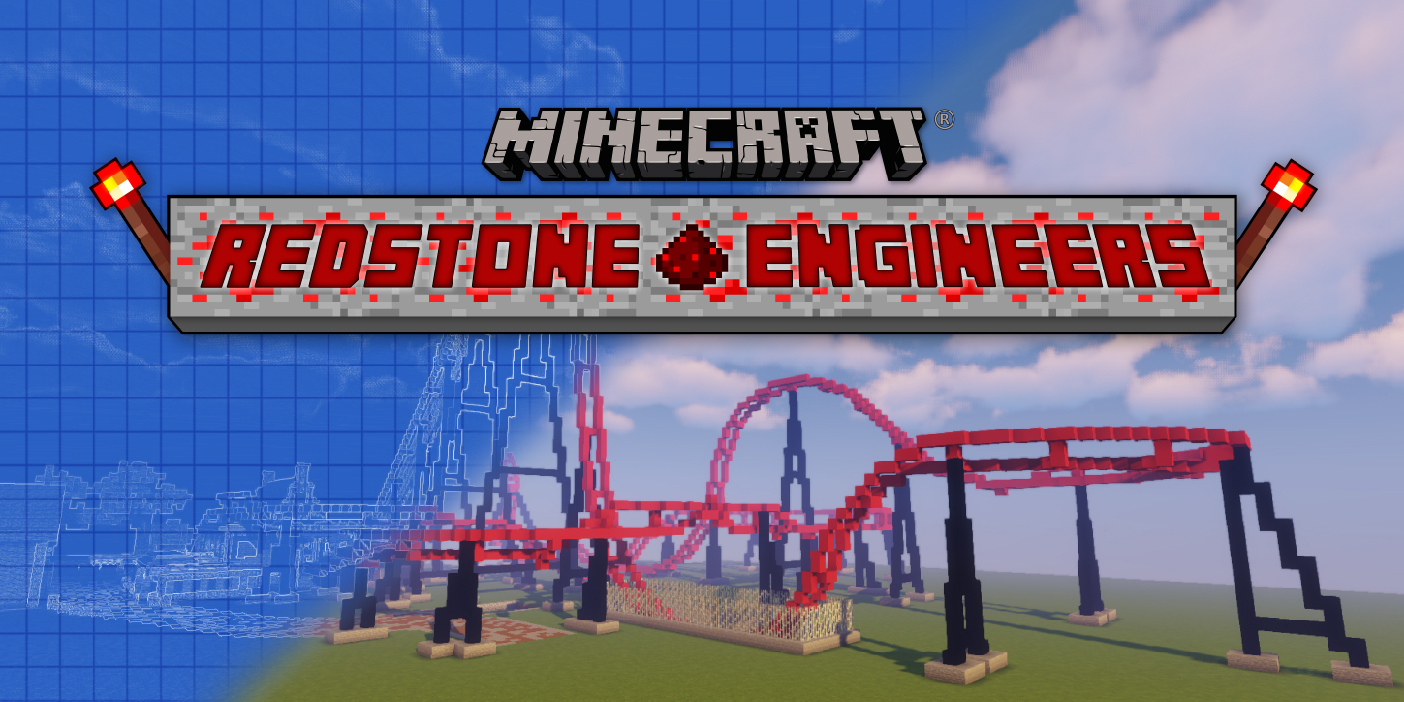This computer-generated image is themed around "Minecraft Redstone Engineers," prominently featuring the iconic Minecraft logo at the very top, complete with a registered trademark symbol. Beneath the logo is a 3D-rendered sign reading "Redstone Engineers" in a bold, pixelated red font, flanked by digital flames extending to the left and right, adding a dynamic touch to the design.

Central to the image is a striking illustration of a red rollercoaster, constructed from Minecraft's signature building blocks. The rollercoaster, supported by black stilts, occupies the right half of the image and is depicted in vivid detail against a vibrant backdrop of green, pixelated grass under a bright blue sky dotted with white clouds. The scene captures the essence of the Minecraft world, emphasizing the game's characteristic blocky aesthetics and pixelated textures.

Splitting the image diagonally, the left half transitions into a blueprint mode, which overlays a darker blue grid with white line drawings of the same rollercoaster. This blueprint section highlights the step-by-step engineering process, from conceptual design to completed build, showcasing the meticulous planning involved in creating complex structures within the game. The blueprint includes detailed annotations and grid lines, further accentuating the technical aspect and the craftsmanship of the Redstone engineers. The entire composition effectively illustrates the journey of turning a creative blueprint into a tangible in-game structure, celebrating the ingenuity and skill of the Minecraft community.